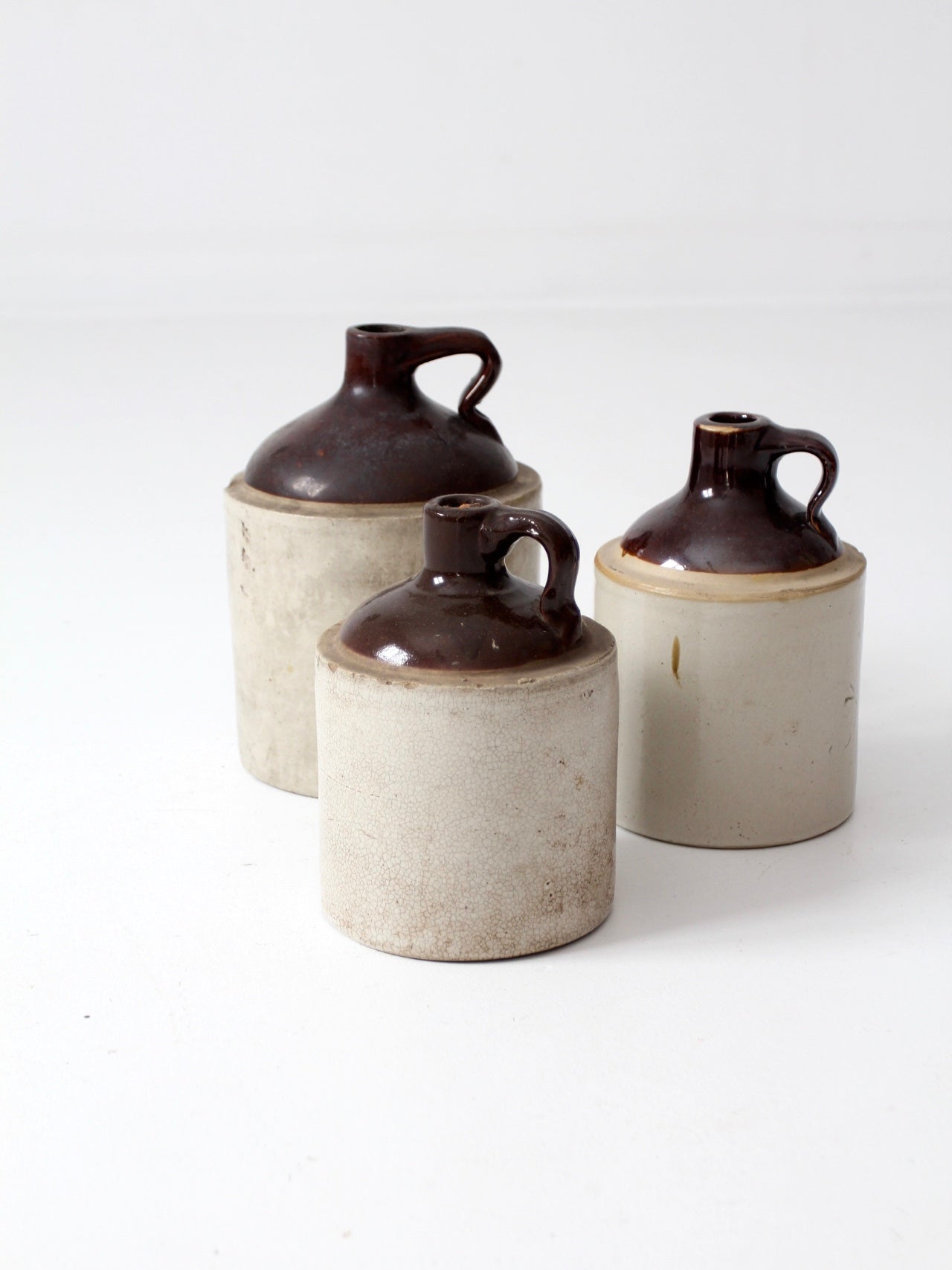This image showcases three vintage moonshine jugs, professionally photographed against a solid white background that offers no depth perception, enhancing the aged aesthetic of the objects. The pottery items feature a unique design with circular, columnar bases extending upward and transitioning into darker brown, bottle-shaped tops, reminiscent of traditional moonshine jugs. The bases are a cream or light tan color, suggesting a cement-like material contrasting with the darker upper portions. Arranged in a triangle formation, the two nearly identical smaller jugs sit in front of the slightly larger one. All three jugs display weathering, adding to their rustic charm, with one jug particularly marked, hinting at their storied pasts.